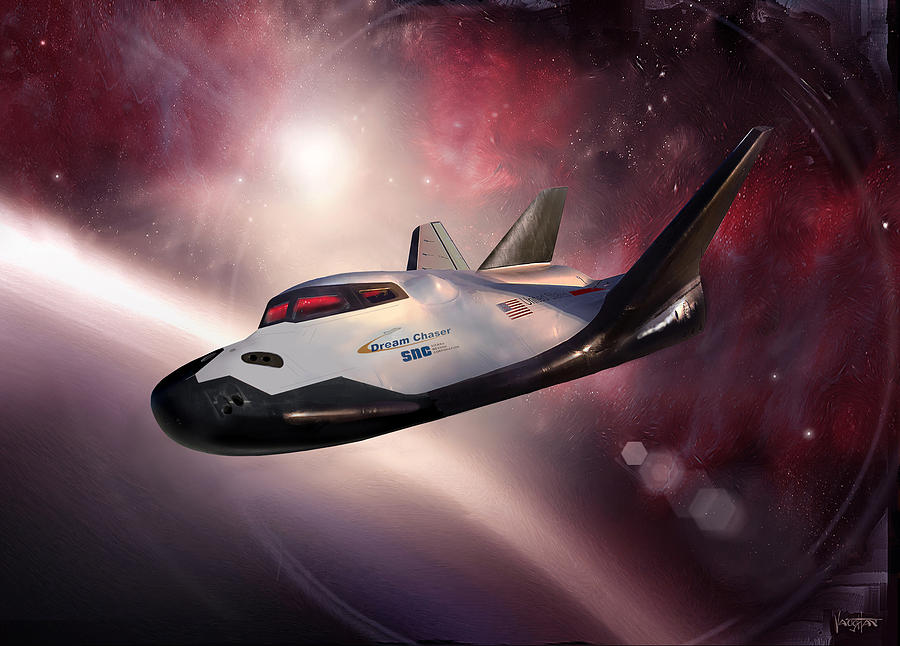This image captures a dramatic scene set in the depths of space, dominated by a prominently featured spacecraft named Dream Chaser SRC. The spacecraft displays a sleek design with a stark contrast between its white upper body and black underbelly, which serves as an ablative shield for re-entry. The vessel has upward-angled wings and a distinctive tail structure. The windows of the cockpit emanate a glowing red light, hinting at intense heat or atmospheric reentry.

The side of the shuttle proudly reads "Dream Chaser SRC," adorned with an American flag and accompanied by the words "United States" in blue, underlined by a gold boomerang-shaped swoosh logo. The spacecraft is captured in sharp detail, contrasting sharply with its blurred, rippled surroundings, suggesting it may be depicted undergoing warp travel or another form of space-time distortion.

The background is a celestial canvas of black space with swirling red and pink nebula-like clouds. A bright band of white light and star speckles suggest a galaxy or another astronomical entity. Towards the top left of the image, the distant Sun casts a subtle glow, adding to the overall ethereal ambiance. In the lower portion of the frame, the immense, curving horizon of what might be a planet suggests a view from orbit, grounding the surreal scene in a semblance of reality.